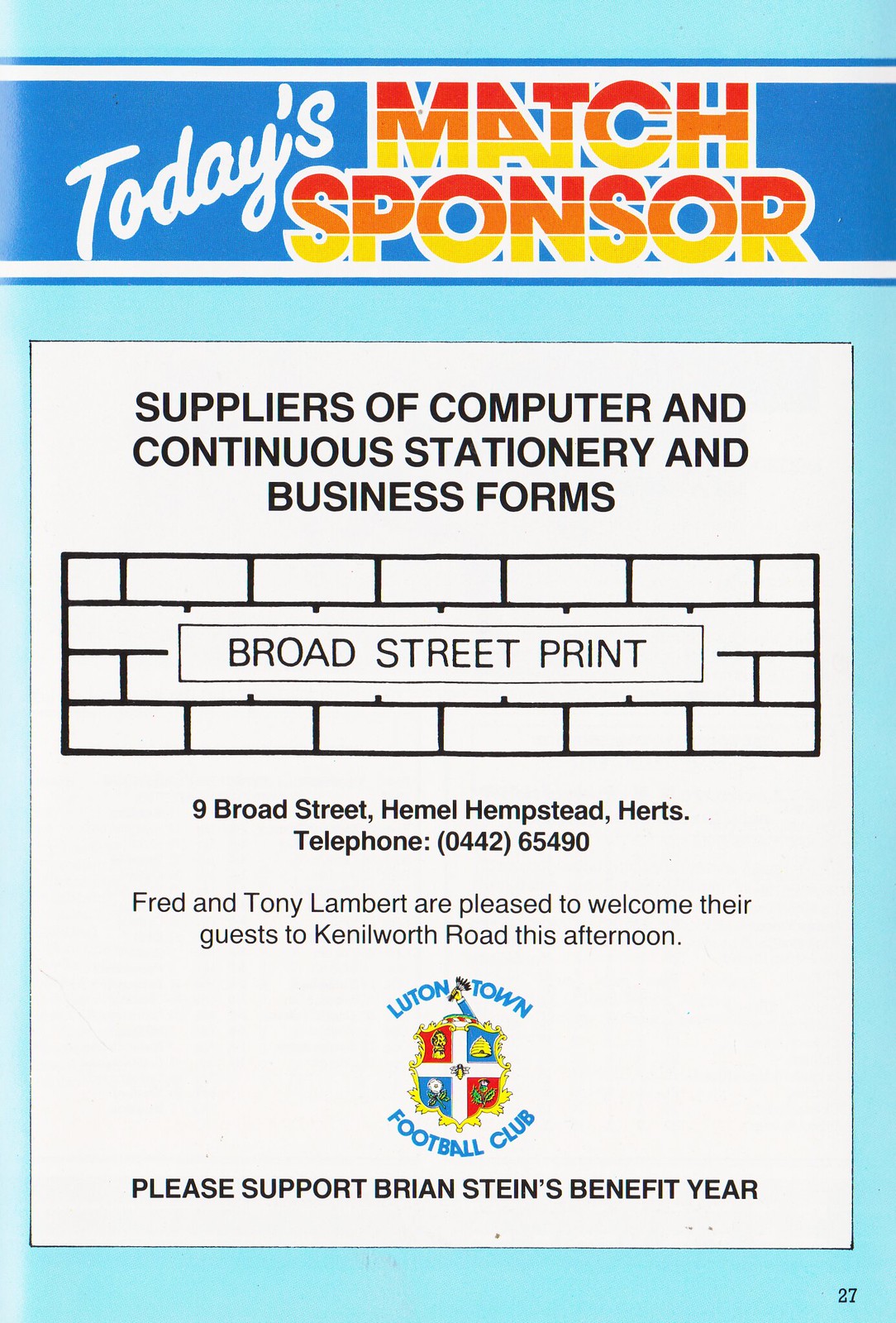The drawing appears to be an advertisement with a light blue background. At the top, there is a dark blue banner with the text "Today's Match Sponsor." The word "Today" is written in a white, stylized, cursive font, slightly diagonal, while "Match Sponsor" is much larger, bold, and features horizontal bands in red, orange, and yellow, making it stand out. Below this, a white rectangle contains the text "Suppliers of computer and continuous stationery and business forms" in black. Further down, there is a graphic of a brick wall with "Broad Street Print" superimposed on it. The address reads "9 Broad Street, Hemel Hempstead, Herts," followed by the telephone number "04442-65490." The image also mentions that "Fred and Tony Lambert are pleased to welcome their guests to Kenilworth Road this afternoon." At the bottom, there is a logo for the Luton Town Football Club, featuring a shield or coat of arms. The final text encourages support for "Brian Stein's benefit year."